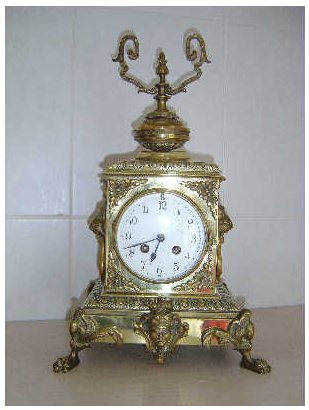The image depicts an ornate, antique clock crafted from what appears to be brass. The clock stands on clawed feet and features a richly decorated rectangular base with horizontally aligned long sides. Above the base sits the clock, encased in a matching decorative brass box. The clock face is white, displaying numbers 1 through 12 in a traditional circular arrangement. The time shown indicates approximately 6:42, with the shorter hour hand positioned between 6 and 7, and the longer minute hand just past the 8. The top of the clock is crowned with an elaborate design, including a spherical element, from which a pointed finial and two antler-like decorative brass extensions emerge. The entire piece is adorned with intricate details, including ornate faces and complex patterns, emphasizing its vintage and artistic craftsmanship.